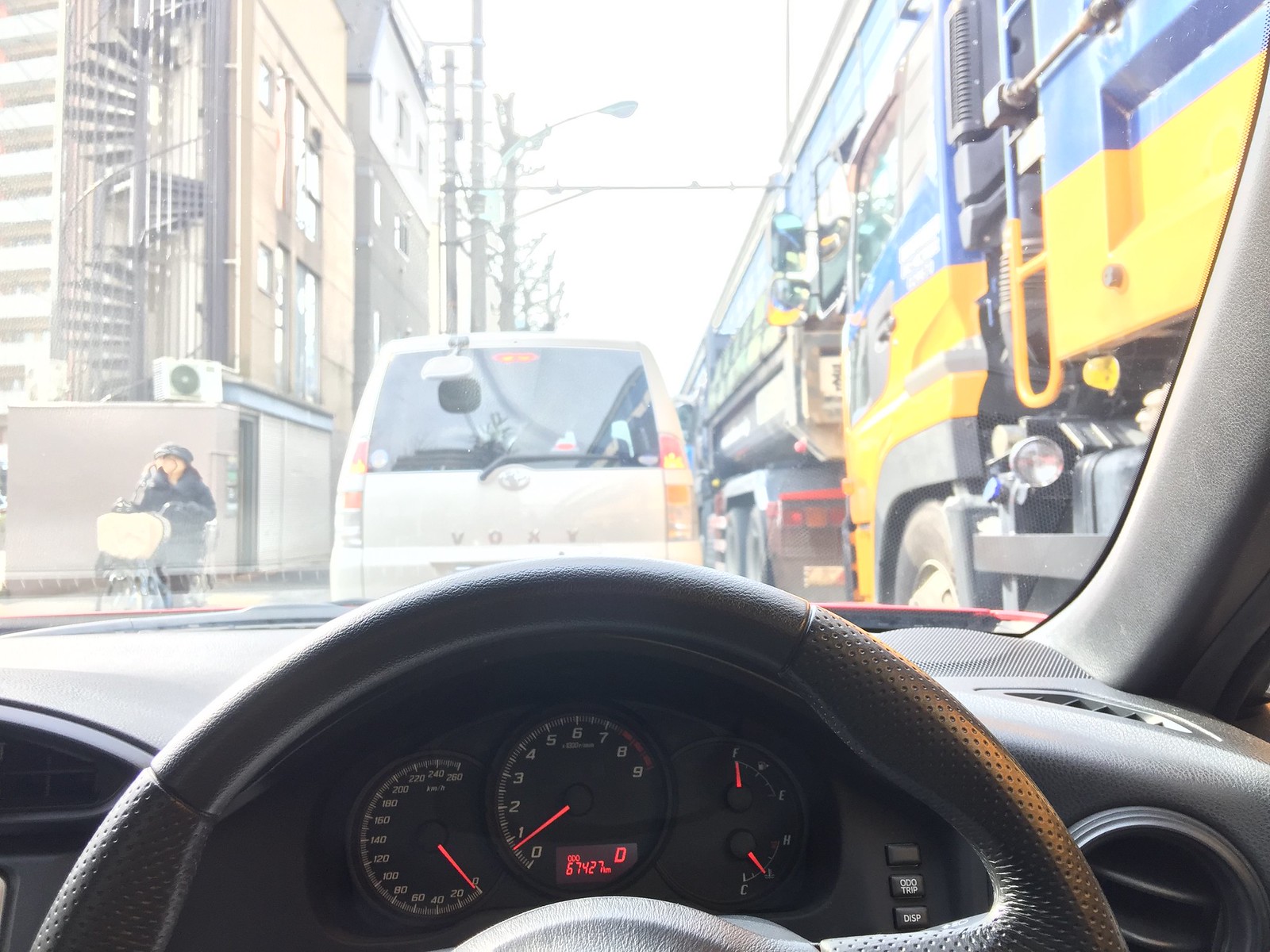The photograph is taken from the driver's seat of a right-hand drive car, showcasing the interior dashboard and a glimpse of the exterior scenery. The top half of the steering wheel is visible, along with the dashboard meters that include a speedometer, currently indicating zero, and a fuel gauge that shows a full tank. The dials are black with white markings for easy readability. Another meter is present in the middle, whose function is unclear and possibly specific to a different country.

Through the windshield, we see a bustling street scene. On the left, a person rides a bicycle, followed closely by a van-like vehicle. To the right, a large dump truck is parked. The street appears narrow, flanked by buildings on both sides. It is daytime, as evidenced by the bright, albeit colorless sky, suggesting either an overcast day or such intense brightness that the sky's hue is washed out. Street lamps line the narrow road, adding to the urban atmosphere.